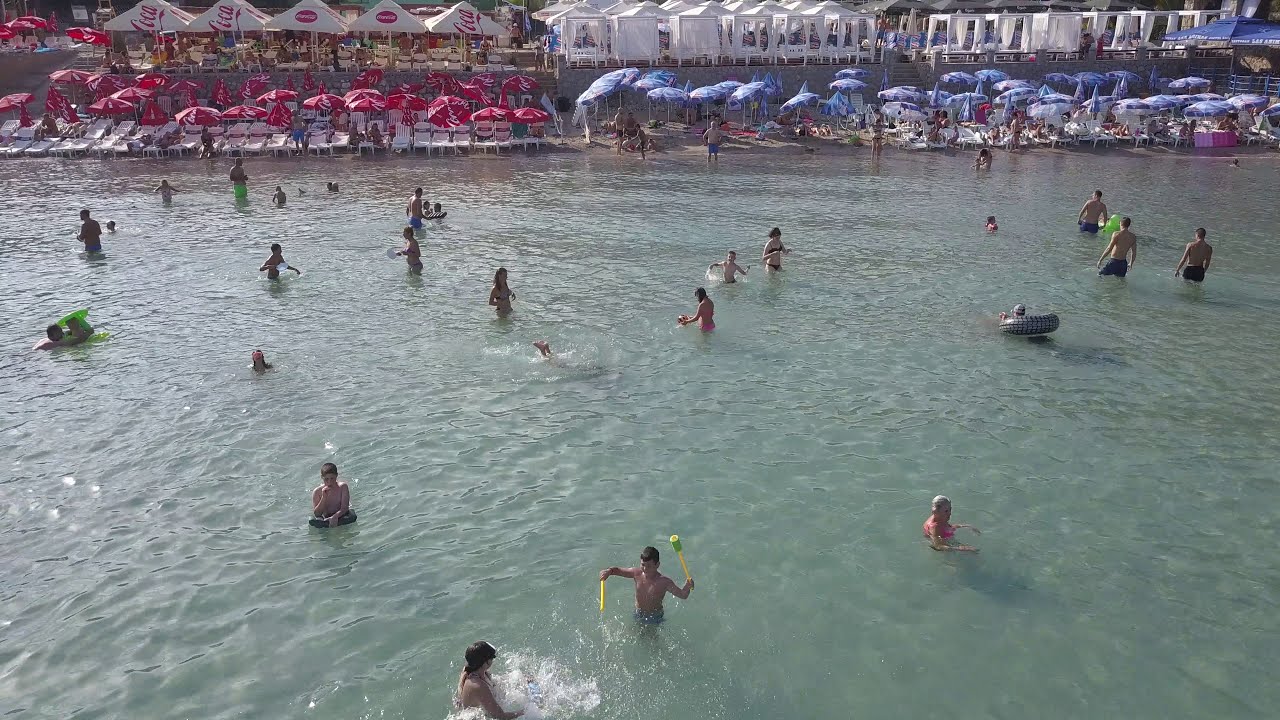This photograph captures a lively beach scene from an elevated vantage point, providing an expansive view of the sea and shoreline. In the upper part of the image, the sandy shore is visible, fringed with red umbrellas to the left and blue umbrellas to the right, creating a clear visual symmetry. Behind these umbrellas, there are tents and kiosks that suggest facilities for dining and other beachside activities. The vast sea dominates the lower portion of the image, its water a slightly greenish hue. Scattered throughout the water are many people enjoying various activities. Some are bathing, while others appear to be learning to swim or playing with rubber hammers and bowls. Towards the right side of the sea, a person floats in a black and gray striped inner tube, wearing a hat. In the bottom center, a boy with swimming goggles brandishes two yellow sticks, seemingly in a playful stance aimed at another swimmer. The overall atmosphere is one of fun and relaxation, with individuals of all ages swimming, waving, and basking in the enjoyment of the day. The calmness of the water hints that this might be a bay or a calmer part of the sea, enhancing the idyllic setting.